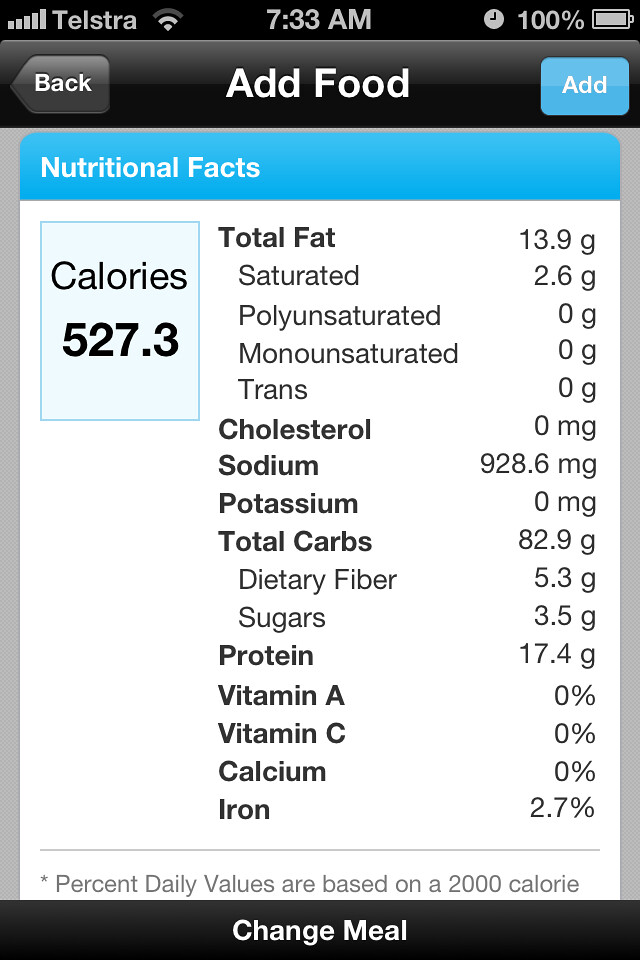The screenshot captures the display of a nutrition tracking app on a smartphone. At the very top, a black border shows essential phone information including network provider "Telstra", the Wi-Fi status, the time "7:33 AM", an alarm clock icon, and a fully charged battery indicator at "100%". Below this, another black bar features three buttons: a "BACK" button in black with white lettering on the left, an "ADD FOOD" prompt in the center, and an "ADD" button in blue with white lettering on the right. 

Underneath a blue bar labeled "NUTRITIONAL FACTS" lies a comprehensive list of nutritional data in white text: 
- Total Calories: 527.3
- Total Fat: 13.9 grams (including Saturated Fat: 2.6 grams, Unsaturated Fat: 0 grams, Monounsaturated Fat: 0 grams, Trans Fat: 0 grams)
- Cholesterol: 0 milligrams
- Sodium: 928.6 milligrams
- Potassium: 0 milligrams
- Total Carbs: 82.9 grams
- Protein, Vitamin A, Vitamin C, Calcium, and Iron listings

At the bottom, a note in black text explains that the percentage daily values are based on a 2,000-calorie diet. Finally, a black bar at the bottom of the screen with white lettering invites users to "CHANGE MEAL".